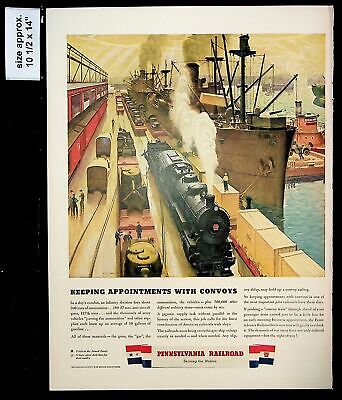This is an old magazine page, approximately 10.5 by 14 inches, featuring a black-bordered square photo inset against a white background. The photo depicts two trains, one of which is black, stationed alongside a large shipping vessel with people on both sides, possibly loading or unloading the train and other cargo. In the background, a body of water with boats can be seen. Underneath the image, there's a title, "Keeping Appointments with Convoys," followed by an article in three columns of small, hard-to-read text. At the bottom center of the page, there's the "Pennsylvania Railroad" banner accompanied by two small flags.